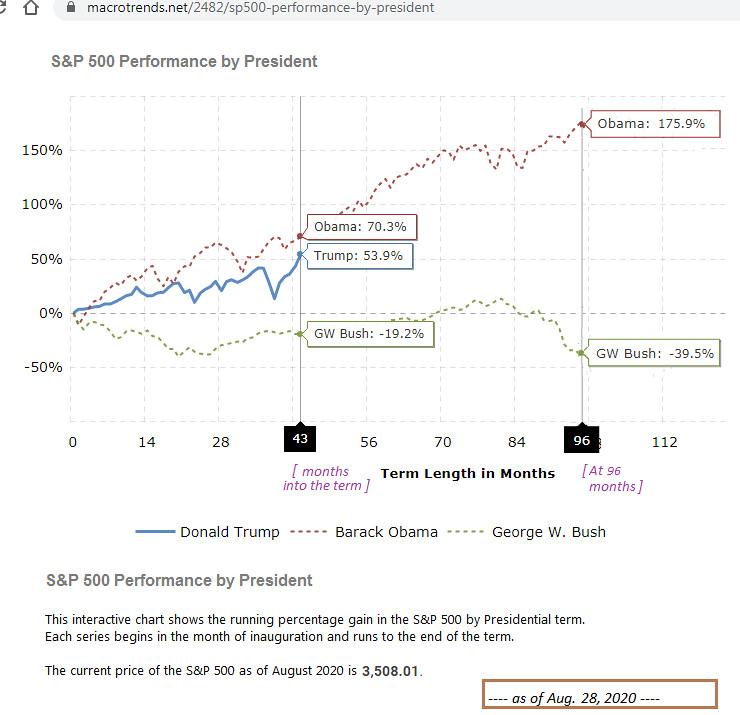The image depicts a detailed chart titled "S&P 500 Performance by President," sourced from the website Macrotrends.net. The chart showcases the stock market performance under three U.S. presidents: George W. Bush, Barack Obama, and Donald Trump. The background is white with various labels and annotations in both black and purple fonts. 

At the top, there's a navigation bar featuring a lock symbol, an up arrow, the website link "macrotrends.net/2482/SP500-performance-by-president," and the text "S&P 500 Performance by President" in gray font. 

The chart itself plots "Term Length in Months" on the horizontal axis, marked at intervals of 0, 14, 28, 43, 56, 70, 84, 96, and 112 months. The vertical axis, labeled in black, ranges from -50% to 150%, indicating the percentage change in the S&P 500 index. 

Three distinct lines represent the different presidencies: a solid blue line for Donald Trump, a red dotted line for Barack Obama, and a green dotted line for George W. Bush. Each line highlights key performance milestones. Bush's performance is noted as -19.2% at 43 months and -39.5% at 96 months, Obama's at 70.3% and 175.9% for the same intervals, and Trump's at 53.9% at 43 months. 

At the bottom of the chart, there is a key alongside the text "S&P 500 Performance by President" which further explains that each series begins at the inauguration month and ends at the term's conclusion. The data is marked as current up to August 28, 2020, when the S&P 500 index stood at 3,508.01. Annotations are in varying colors to denote each president's data points, ensuring clarity and visual distinction.